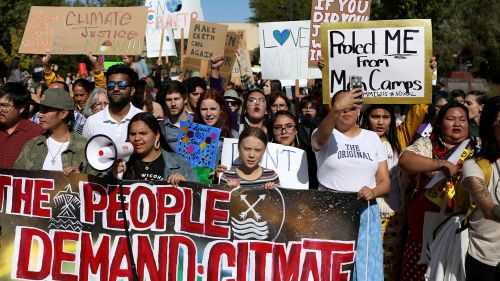In this vibrant, full-color photograph taken on a sunny day using natural light, a large crowd of climate change protesters is gathered outdoors. The image, horizontally rectangular with no specific border, prominently features Greta Thunberg at the center, recognizable by her youthful appearance and pulled-back hair, as she looks directly into the camera. Flanked by activists, she holds part of a banner that reads, “The People Demand Climate” in bold red letters with a white outline. To Greta's left, a Hispanic woman wields a megaphone, and to her right, another woman is captured mid-photo with her phone. The diverse crowd behind them holds various signs, some clearly legible with phrases like "Climate Justice," "Make Earth Cool Again," and "Love," while others are partially obscured or washed out. The banner appears stylized with Native American imagery, possibly depicting an eagle, arrows, and water. The background features a blend of black and orange hues, contributing to the striking visual of the starry night sky and adding depth to the scene.